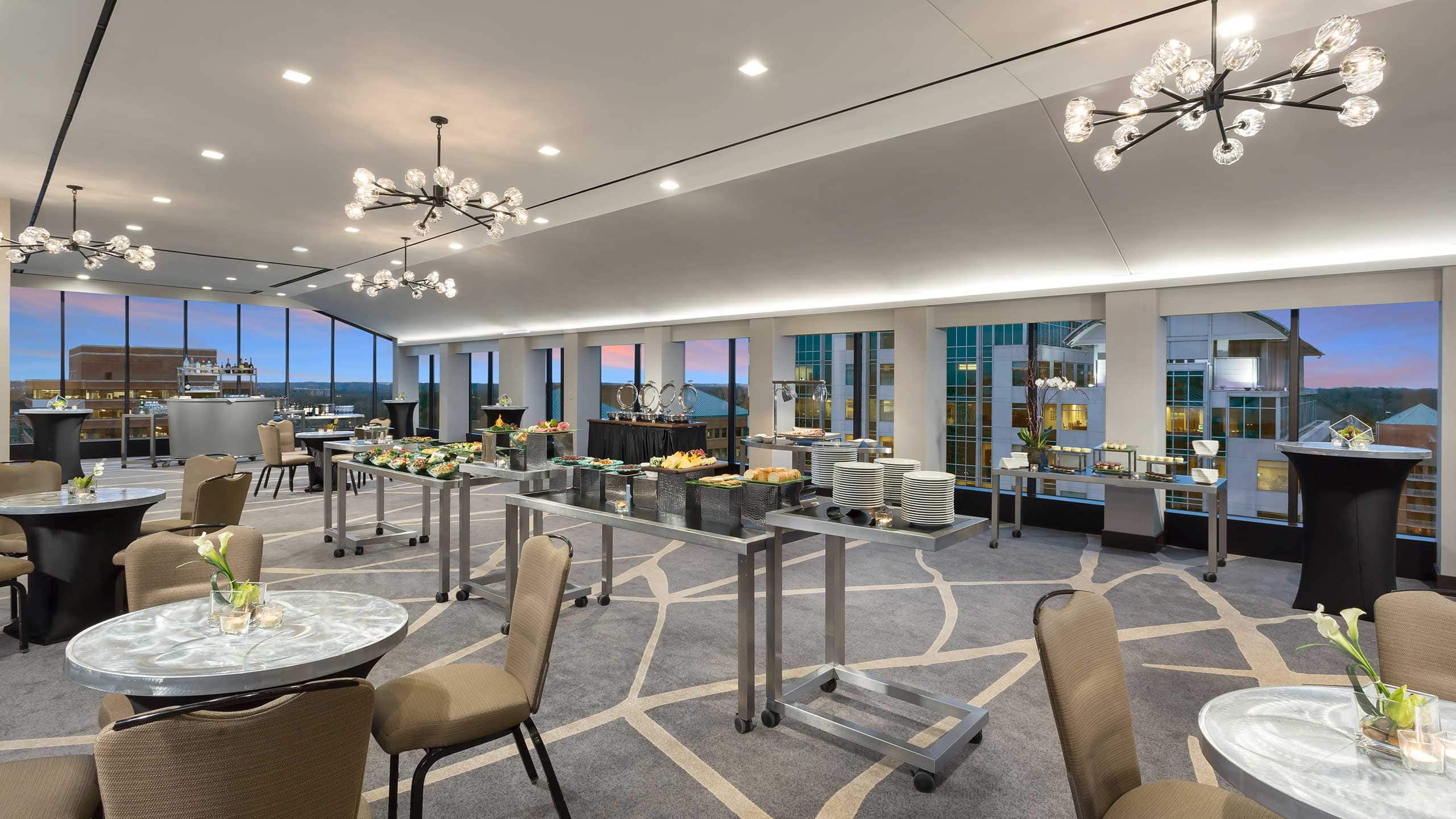The photograph depicts an elegant, high-level dining area, likely a high-rise restaurant, set during the twilight hours, showcasing a purple-pinkish and blue sky through large windows. The room features modern, ornate decor with brightly lit ceiling lamps, including distinctive chandeliers composed of series of hanging balls. Below, a long central buffet table, lined with food and multiple metal containers, dominates the space. Surrounding it are several round tables with stone-like off-white tops and brown chairs. Green foliage adorns each table, adding a touch of nature to the modern setting. The carpet is grey with a design resembling white stripes or lines, contributing to the sophisticated ambiance. The area beside the windows also includes taller standing tables for casual dining. The overall impression is of a contemporary, well-appointed restaurant designed for a high-end dining experience.